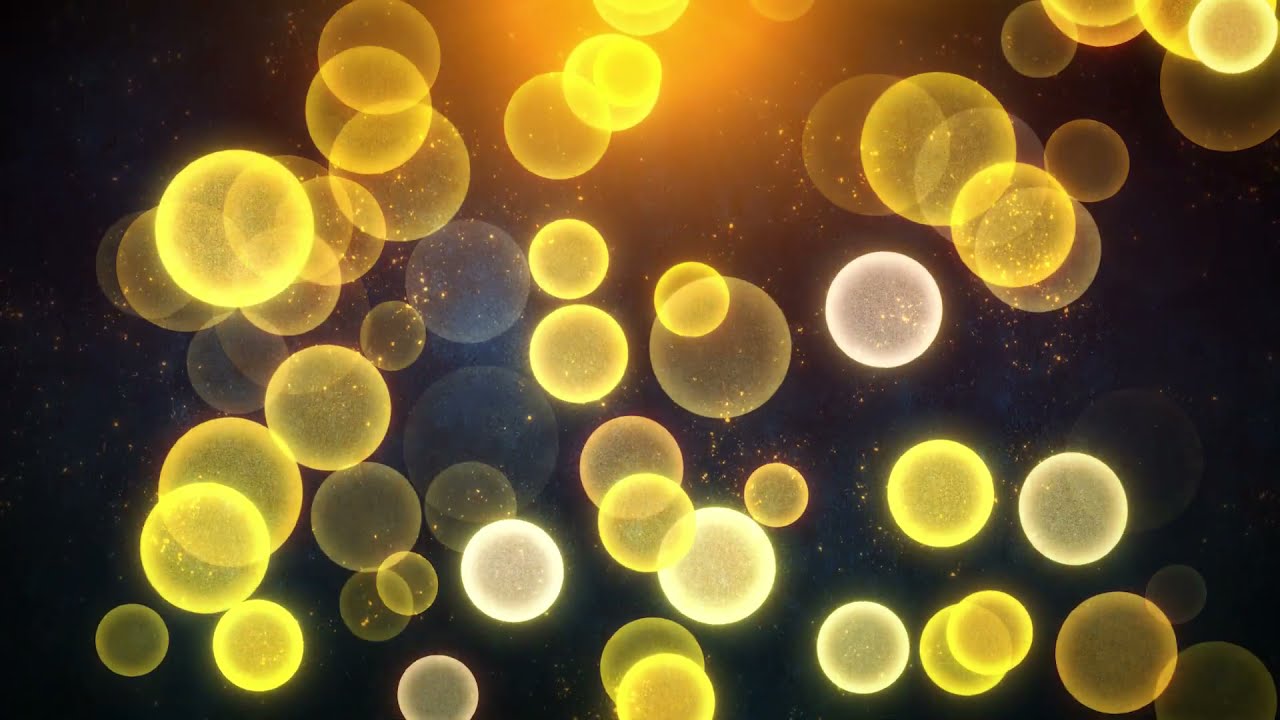The image presents a captivating computer-generated artwork set against a deep black background, reminiscent of a night sky. The scene is filled with an array of semi-transparent bubbles or spheres of varying sizes, some appearing large and others small, creating a sense of three-dimensional depth. These spheres are scattered across the composition, floating in different directions. They exhibit a range of colors and luminosities, including warm yellows, glowing golds, whites, and some cooler blues. The transparency of the spheres allows them to overlay each other, further enhancing the depth effect. Bright, star-like yellow specks dotted throughout the background contribute to the celestial theme. At the very top center of the image, a bright yellow-orange light, reminiscent of the sun, shines with a golden hue, adding a focal point of illumination. The combination of these glowing spheres and the starry backdrop creates a harmonious and visually striking composition.